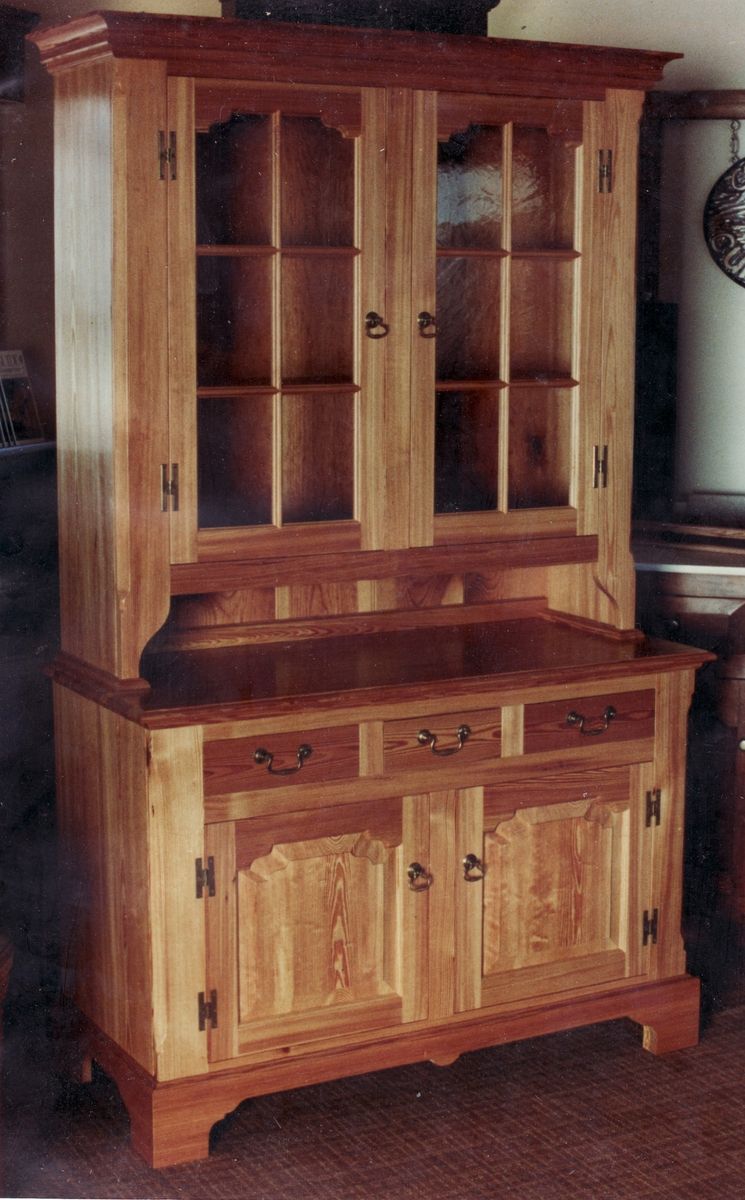This portrait-oriented, color photograph captures a wood china hutch or cabinet positioned in a home setting against a white wall. The image quality is slightly grainy, suggesting it was taken with an older camera. The cabinet, constructed in photographic realism style, showcases various shades and textures of brown wood, predominantly in a honey gold and darker brown palette.

At the bottom, the piece features two large doors with round pulls in the center and brass hinges on both sides, encompassing two-thirds of the cabinet’s height. Above these doors are three horizontal drawers equipped with hanging handles. A flat surface separates this lower section from the upper hutch, which is enclosed by two arched doors with glass panels. The upper doors meet in the center, each adorned with brass door pulls and hinges. The top of the cabinet is finished with a decorative molding. Each segment of the wooden structure displays a distinct combination of light and dark brown shades, contributing to its detailed and rich visual appeal. Despite the slightly elevated angle from right to left, the craftsmanship of this wooden furniture piece remains evident and charming.